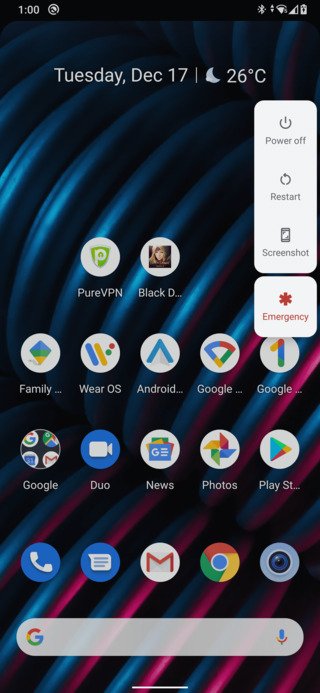The home screen of the cell phone displays a variety of details and features. It is currently 1 o'clock, with the time indicated at the top left of the screen. On the right side, we see that notifications are silenced, and the battery level is approximately 20%. There are 2-3 bars of signal strength available. 

At the very top of the screen, in white text, the date and temperature are shown: "Tuesday, December 17th," with the temperature at 26 degrees Celsius. A crescent moon icon also appears next to the temperature, indicating nighttime or a specific mode involving the moon phase.

The background of the home screen features a visually striking wallpaper of a metal coil on a black backdrop. The coil starts off as blue and transitions to magenta and gray as light reflects off of it, creating a dynamic and appealing effect.

At the bottom of the screen sits a Google search bar with a microphone icon to the right, facilitating quick searches and voice commands. Below the date and temperature, there are options for power off, restart, screenshot, and emergency functionalities.

The home screen is populated with various widgets and app icons, including PureVPN, Family, Wear OS, Android, Google, another Google widget, Duo, Google News, Photos, and PlayStation. There are also icons for calling, texting, Gmail, Chrome, and an unrecognized application.